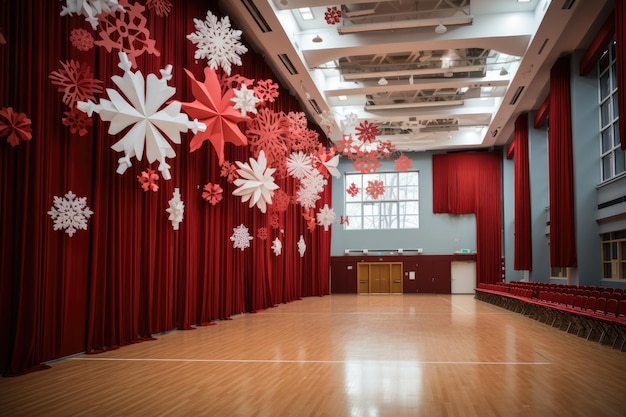The image depicts a large, elaborately decorated room, possibly a school auditorium or gymnasium, with high ceilings and polished hardwood floors resembling a basketball court. The space is designed for a special event, featuring numerous large red curtains that stretch from floor to ceiling, complementing tall, vaulted windows and wooden doors with multiple panels. The right-hand side of the room houses rows of red folding chairs, lined up from one end to the other. Hanging from the ceiling are dozens of massive, decorative red and white snowflakes, each measuring about five to six feet across, creating a festive atmosphere. Visible HVAC systems are mounted high on the ceiling, ensuring ample lighting and ventilation throughout the space. The overall scene suggests a setting prepared for a dance, performance, or party, showcasing a meticulous and festive decoration effort.